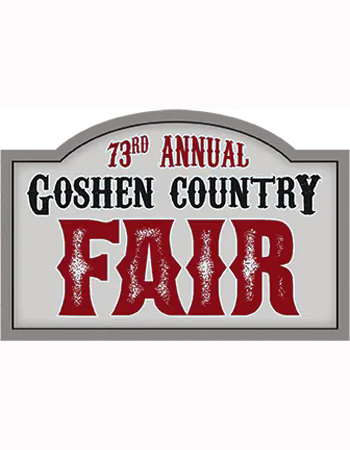In the image, a prominent banner announces the 73rd Annual Goshen Country Fair. The banner, shaped like a trapezoid with a domed top reminiscent of a house, features a mostly gray background with the top portion in white. The entire sign is bordered by a gray line, followed by an inner thin black line that frames the content neatly.

The text on the banner is formatted with all capital letters. The phrase "73RD ANNUAL" is prominently displayed in bold red font, with the 'R' and 'D' as superscripts. Below this, "GOSHEN COUNTRY" is written in larger black letters, providing a strong contrast. The word "FAIR" is the most emphasized, rendered in large, bold red font with white dots enhancing each letter, making it strikingly visible.